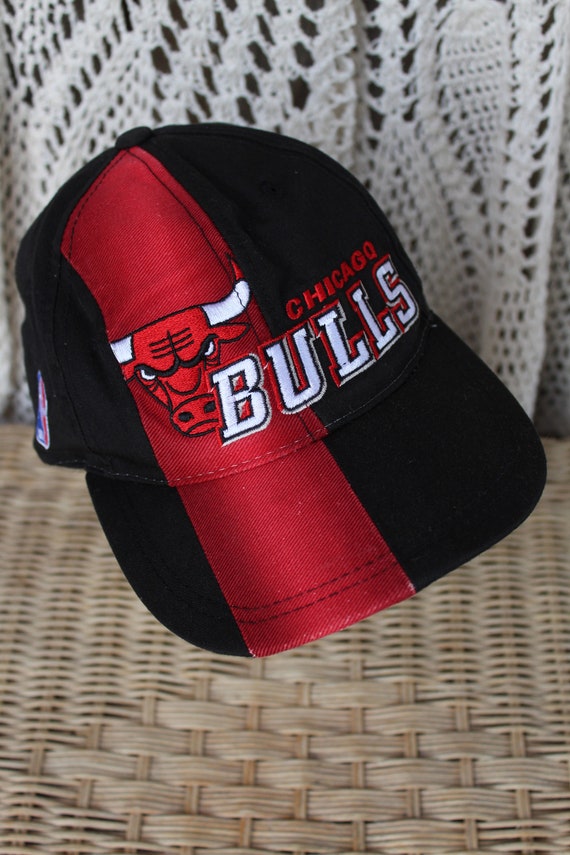The photograph, taken indoors, captures a black baseball cap prominently featuring the iconic Chicago Bulls logo. The cap has a bold red stripe running from the center top down through the brim, housing a red bull with white horns and white eyes. Just to the right of the bull, "Chicago" is stitched in small red letters, while "Bulls" is emblazoned in larger white letters outlined in black below. The cap rests at an angle on a woven wicker chair, characterized by its light tan color and a basket-style weave with a thicker central pattern and smaller gaps around the edges. Draped over the back of the chair is a delicate, white crocheted blanket or shawl that enhances the cozy, indoor setting of the scene.